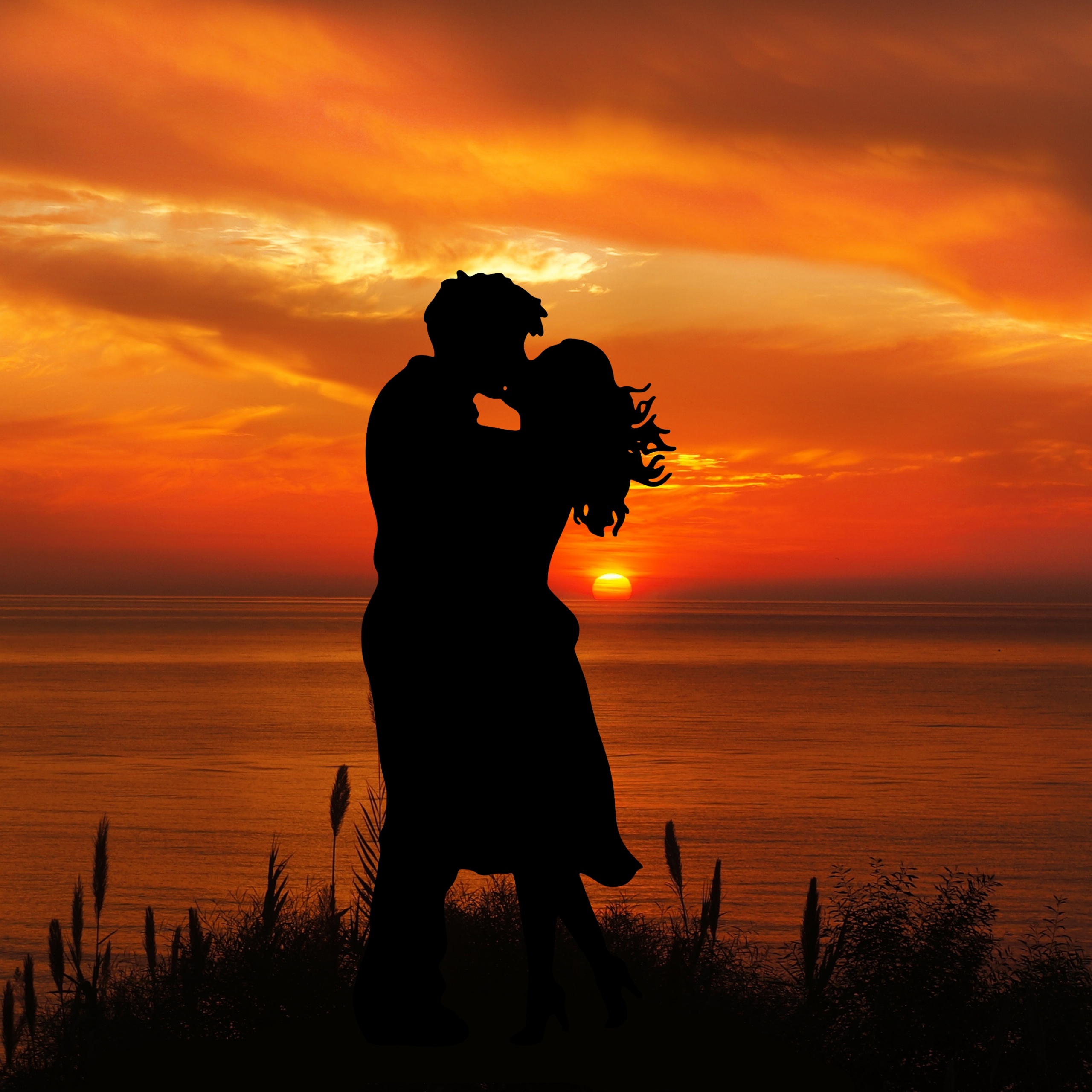This highly detailed and quality-edited image captures a touching moment of a couple kissing at sunset. The couple appears as black silhouettes, one taller with short hair and the other slightly shorter with long hair blowing in the wind, who tips her head back to kiss. They stand embraced on a grassy shoreline, with some weeds poking up from the ground. The background is a stunning sunset over the ocean, with the horizon placed halfway up the image. The sky is a vivid blend of oranges, yellows, and reds, with clouds scattered, and the sun setting into the calm water. The specific sharpness and artistic style of the couple's silhouettes, particularly in details such as the animated appearance of the hair, suggest they were digitally added to the photograph, contributing to the uniqueness and emotional impact of the image.